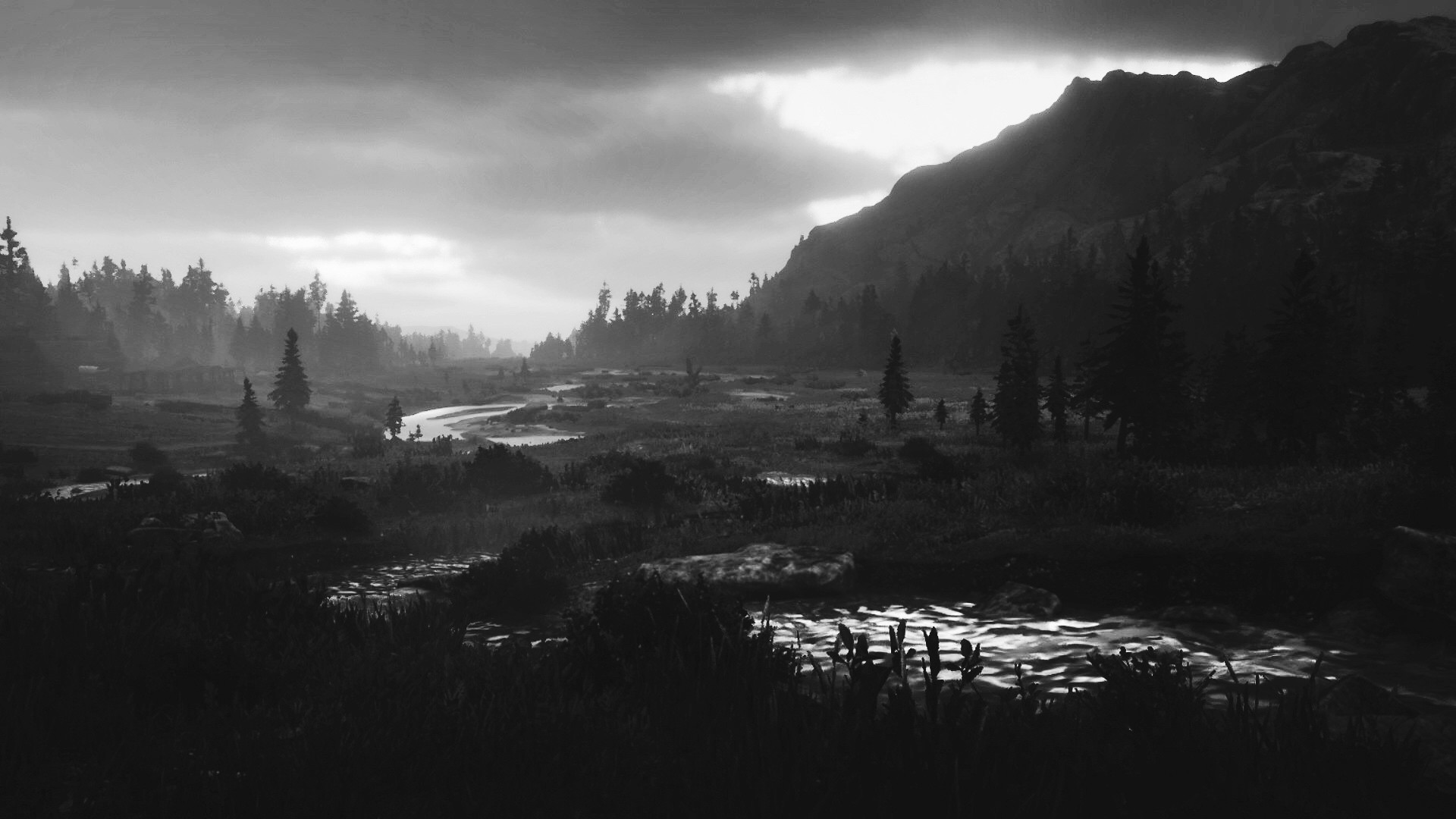A black and white image captures a serene natural landscape, reminiscent of a vintage photograph. The top left-hand corner is filled with ethereal clouds, accentuated by a bright spot in the upper right, likely the sun. The monochrome palette obscures the true color of the sky, leaving its hue to the imagination. On the right side, imposing dark mountains create a striking contrast against the lighter sky. Beneath the clouds on the left, a dense canopy of trees stretches downward, their foliage merging into the darker tones at the bottom of the frame. The lower portion of the image is dominated by more leaves, their rough and rigid outlines adding texture to the scene. At the bottom right, a body of water reflects the surrounding trees, completing the tranquil, yet dramatic, landscape.